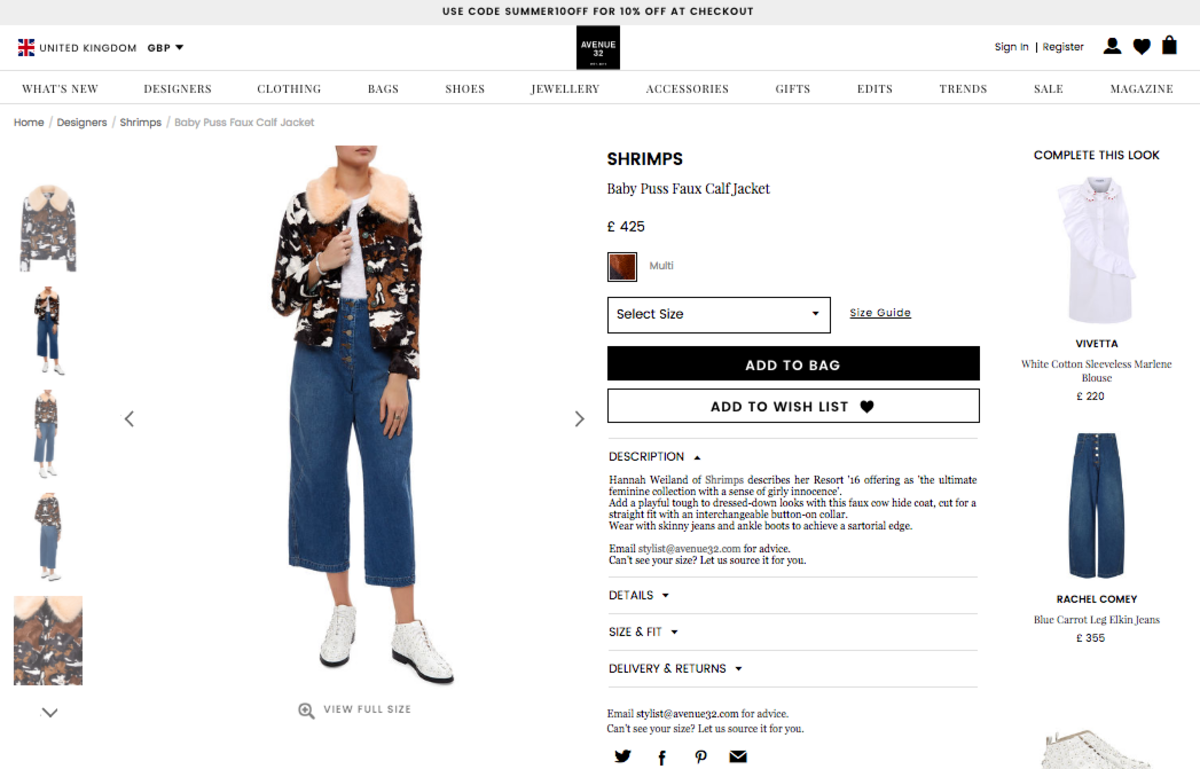The image depicts a webpage from a clothing brand or store named "Avenue 32." The website's logo features a plain black square with the brand name "Avenue 32" written in white font, with "Avenue" on top and "32" below. Though some of the fine print is too small to read, the site prominently displays a promotional gray rectangle at the top, offering a discount: "Use code SUMMER10OFF for 10% off at checkout."

To the left of the Avenue 32 logo, there is an option to select the United Kingdom and a dropdown menu for GBP, the currency for displaying prices. The main menu bar includes categories like What's New, Designers, Clothing, Bags, Shoes, Jewellery, Accessories, Gifts, Edits, Trends, Sale, and Magazine, all written in British English.

The featured product is the Shrimps Baby Puss Faux Calf Jacket. The model is wearing this jacket, characterized by its brown, white, and black pattern with a strawberry tan fur lining. The model also wears a white shirt underneath, short wide-legged jeans, and white wicker shoes with black soles. The jacket is priced at £425, with size selection and a size guide accessible via dropdown menus. Two buttons are available for user actions: a black "Add to Bag" button and a white "Add to Wishlist" button with a heart icon.

Additional descriptions and details about the product can be found in dropdown menus, and there are share buttons for Twitter, Facebook, Pinterest, and Email. Featured alongside the main product are other clothing items like the "Vivetta" white frilly shirt and the "Rachel Comey" broad-legged jeans.